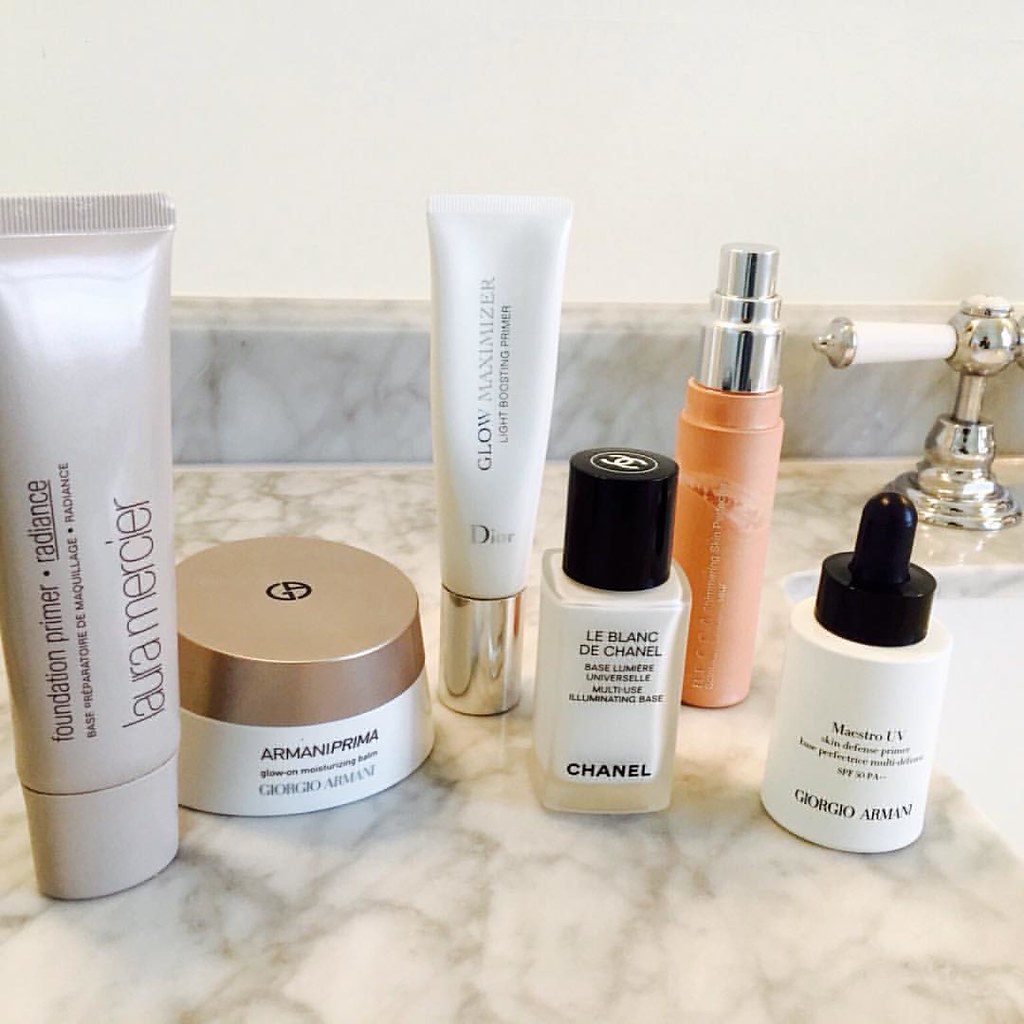This image showcases an elaborate skincare and makeup routine featuring an array of high-end products. On the left side, there is a Laura Mercier Foundation Primer in the variant "Radiant Radiance," housed in a tall tube. Moving to the right, there is a Giorgio Armani Prima Glow-On Moisturizing Lotion, designed to add extra hydration and glow to the skin. In the center-right, a Dior Glow Maximizer is prominently displayed, known for its radiance-boosting properties. Next to it is a smaller tube of Chanel's Le Blanc de Chanel Multi-Use Illuminating Base, which provides a brightening effect. Further to the right, there is an orange spray tube, although the specific brand and product name are not clear. Lastly, on the far right, an elegant Maestro UV by Giorgio Armani can be seen, which likely serves as a protective UV base. This collection demonstrates a commitment to luxurious and high-performance skincare and makeup products.